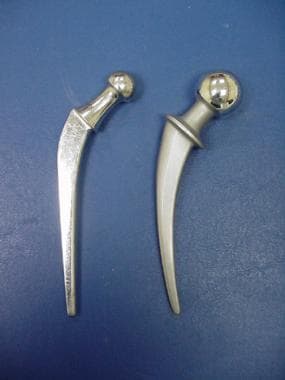This photograph captures two metallic objects placed side by side on a chambray blue fabric background. Both items appear to be crafted from light silver metal, possibly stainless steel. The object on the left features a smaller, rounded knob at the top, transitioning into a cylindrical hilt, and ending in a curved, tooth-like blade with sharp edges. A glint of light reflects off its surface, highlighting its polished appearance. In contrast, the object on the right has a larger, duller round top, followed by a slightly less shiny cylindrical hilt, and a curved blade that is more saber-like, with a rounded yet not sharp bottom edge. Both objects share similar colors and design elements, with subtle differences in size and finish. There are no artist marks or text present in the image, allowing the objects' intricate details and craftsmanship to stand out against the textured blue backdrop.